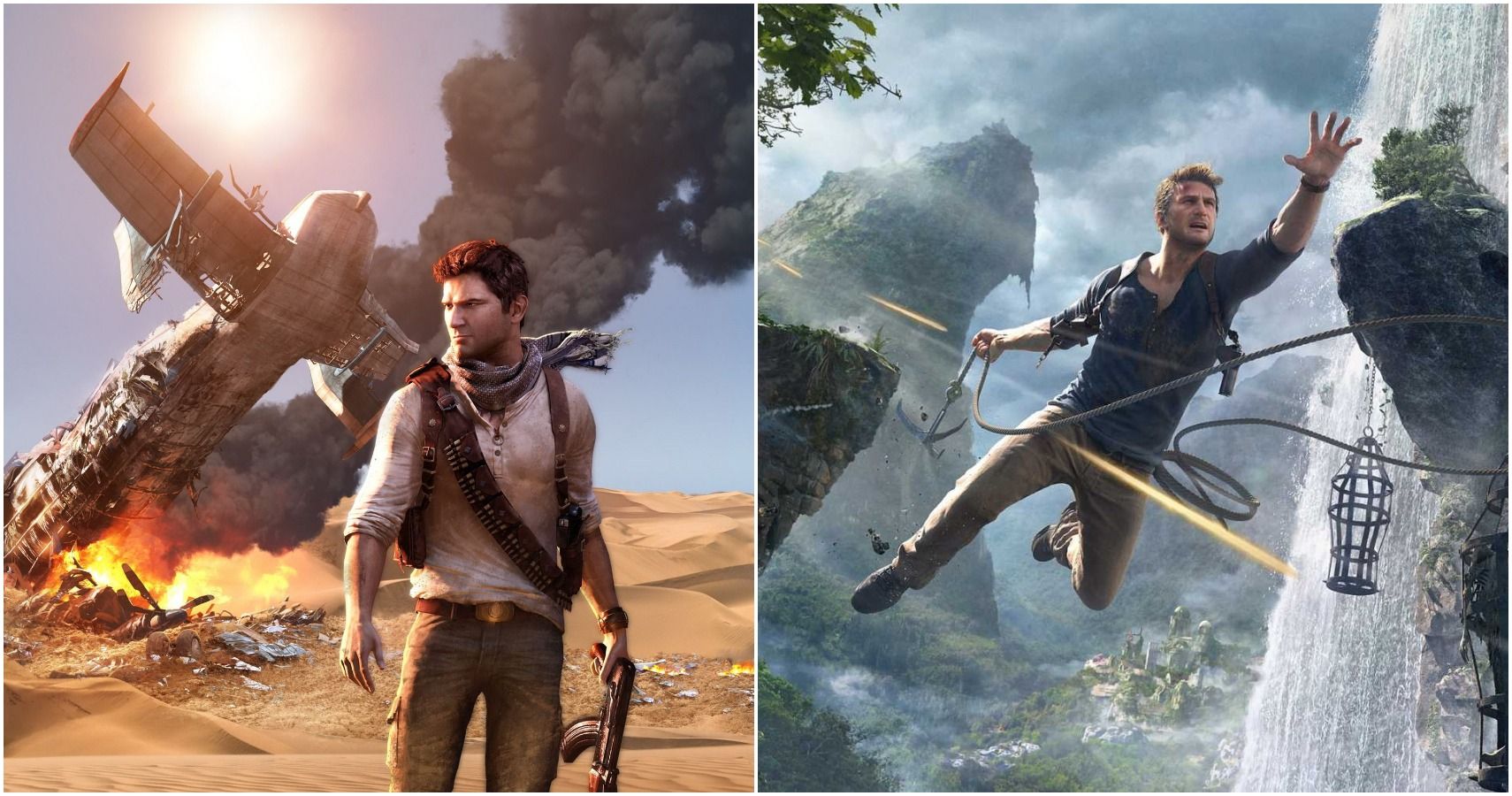A stunning, computer-generated image capturing dynamic scenes resembling video game characters in action. On the left side, a man stands in front of an exploding spacecraft, with striking debris surrounding the area, indicating an intense moment of peril. To the right, another character reaches out towards a rushing white waterfall, the cascading water depicted with remarkable detail, emphasizing its swift and powerful descent. The overall composition showcases impressive AI-generated artistry, highlighting both the realistic textures and the dramatic atmospheres within the scenes.